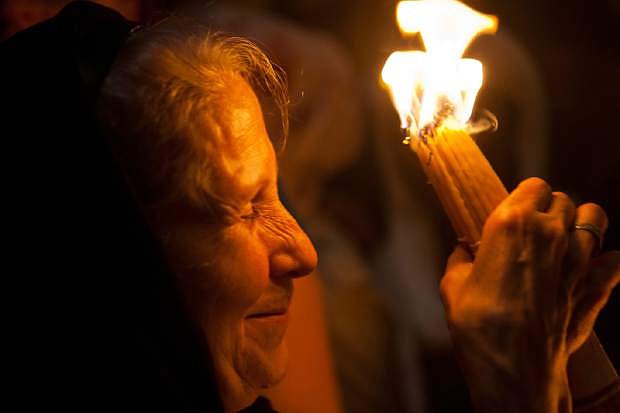The photograph captures the profile of an older person, likely a woman, on the left side of the image. Her thinning, gray hair and pronounced wrinkles around her eyes and nose indicate her age. Her eyes are tightly closed and her mouth is set in a subtle, closed smile, giving her an expression that could be interpreted as peaceful or grimacing. She holds up her right hand, with a simple, thin wedding band visible on her ring finger, clutching a cylindrical object, possibly a wax candle or incense, which emits a large, bright flame. The golden-yellow and orange hues from the flame's light cast an ethereal glow on her face, creating a stark contrast against the completely dark and black background. The photograph evokes a sense of solemnity and devotion, suggesting a possible religious or ceremonial context, though the exact occasion remains uncertain.